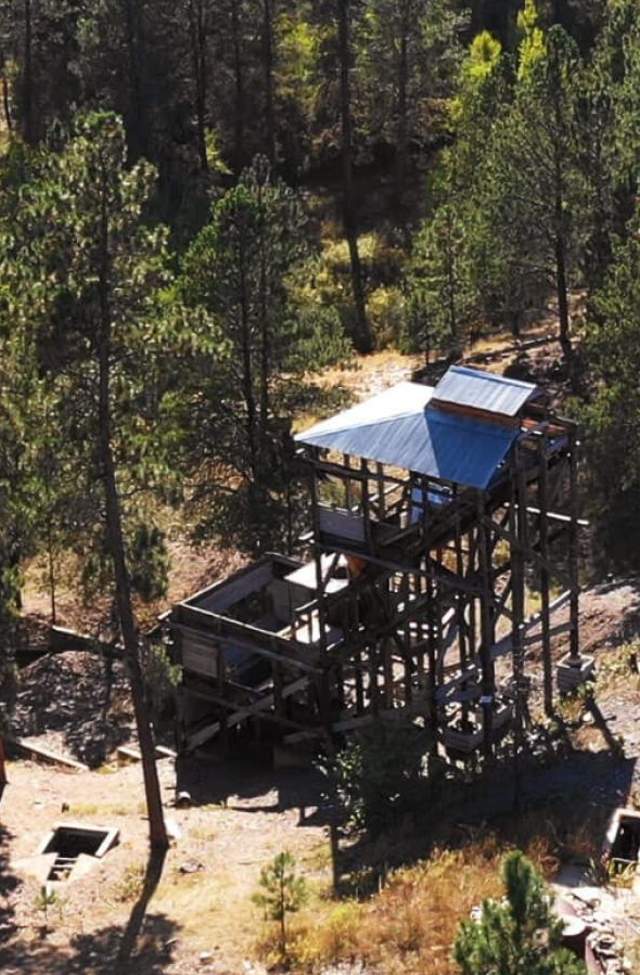This aerial photograph captures a vertically oriented scene of a large wooden platform structure with a metal roof, nestled in a dense forest of tall pine trees. The wooden structure, centrally positioned in the image, features several flights of stairs descending to a larger ground-level building. Adjacent to the elevated platform, there is a smaller roof equipped with solar cells. The surrounding area, thick with green foliage and tall brown tree trunks, indicates a late summer afternoon setting, as sunlight filters through the trees, casting shadows and highlights across the scene. The compound includes a curious square concrete opening with a small grill to the left of a prominent tree, suggesting it might be a part of a forestry station or ranger station. Overall, the image reflects a tranquil, somewhat rugged forest scene, possibly associated with a camping setup, hunting stand, or even a survival bunker.